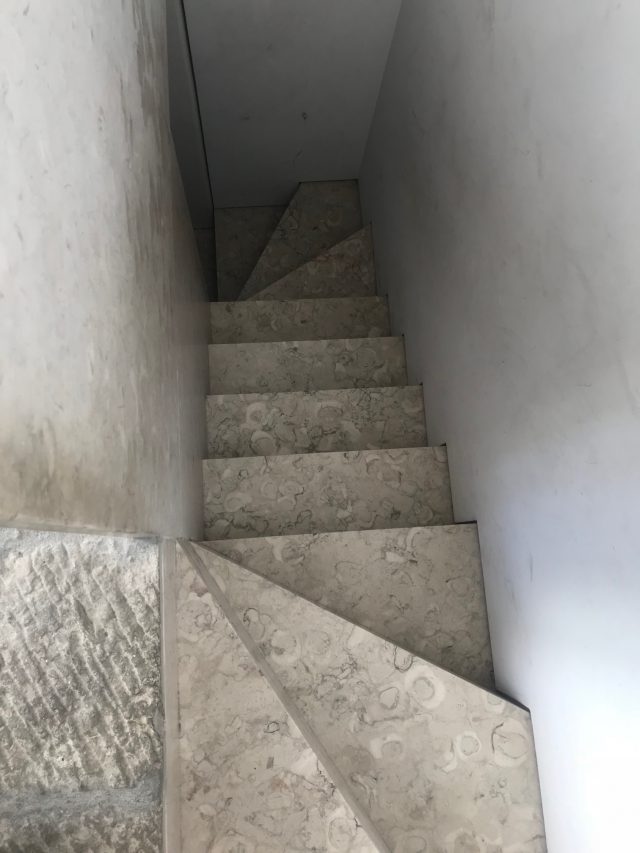The image captures a precipitous view down an exceedingly narrow and steep stairway, characterized by a tight and constrained structure. At the top and bottom, the stairway curves sharply, directing the viewer's gaze downward along the first flight or corner. To the left, a doorway opens onto this cramped passageway.

The walls, rugged and grooved like worn stone, guide the eye to the concrete steps below, which appear almost fossilized with intricate patterns. The first two steps are triangular, winding counterclockwise towards the upper part of the frame, while the third step, though square, is truncated by the second. From there, the stairs transition into four conventional steps descending straight down.

On either side, the plaster walls are oppressively narrow, granting a mere two and a half feet of width. Towards the bottom, three additional steps curve sharply counterclockwise to the left, leading towards another open door.

Dimly lit, the scene relies solely on illumination from the doorway at the top, creating an eerie and foreboding atmosphere. The cramped, poorly lit space accentuates the treacherous nature of the descent, making it evident that navigating this staircase would be exceedingly challenging, particularly when burdened with carrying items.